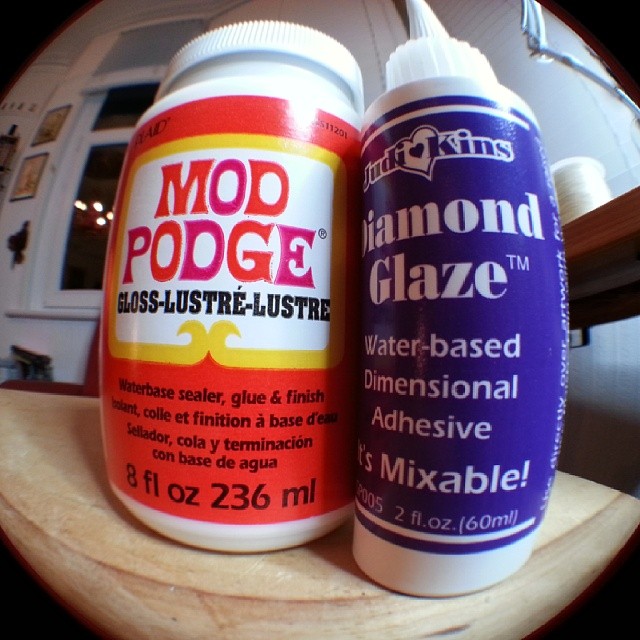The image captures a distorted, close-up view of two craft supply bottles sitting on a table, possibly in a home office. The fisheye lens effect warps the edges, giving the photograph a rounded appearance. In the background, a window is partially visible along with a shelf containing a roll of twine and some hanging pictures on the wall.

The bottle on the left is a white jar with a red label. The label has a prominent white square with a yellow border, featuring the text "Mod Podge" in orange-pink lettering. Below this, black text reads "Gloss Luster Luster" with translations in French and Spanish. Toward the bottom, it states, "Water-Based Sealer, Glue and Finish." This jar holds 8 fluid ounces (236 milliliters) of product.

The bottle on the right is a blue tube with a white cap and a squirt top. The label features the name "Judikins," decorated with a heart symbol in the center, and outlined in white. The product is named "Diamond Glaze," described further as a "Water-Based Dimensional Adhesive" that is mixable. It contains 2 fluid ounces (60 milliliters) of adhesive.

The close-up, distorted perspective, coupled with the clear product details on the labels, emphasizes the utility and branding of these craft supplies amidst a cozy, personal workspace.